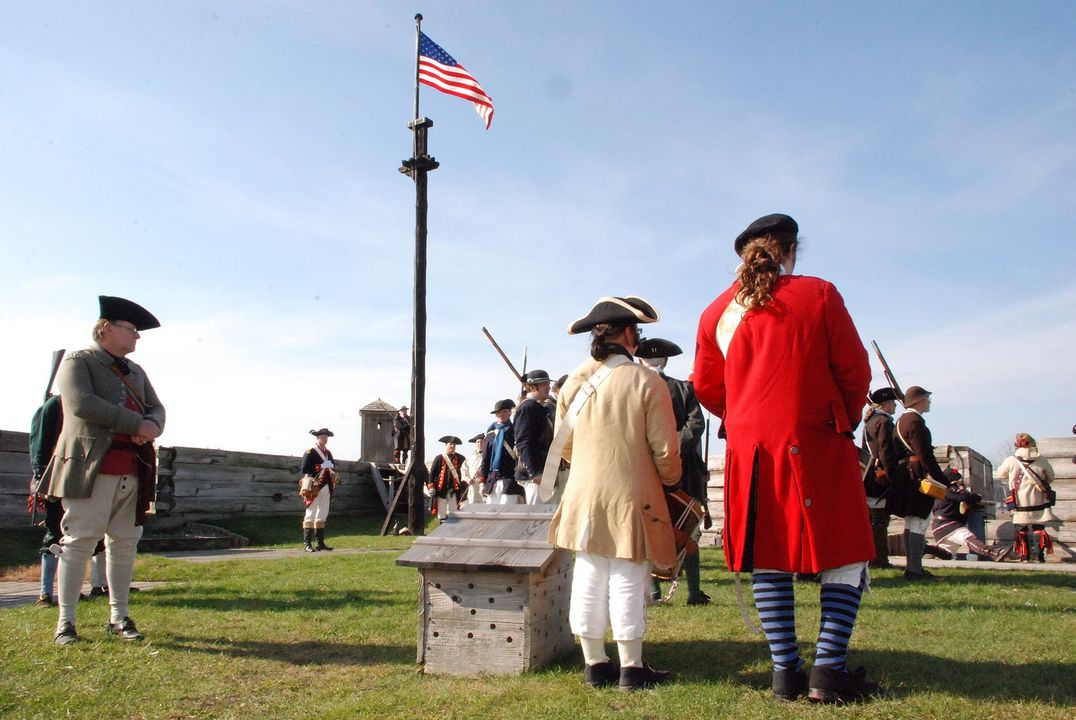In the image, we see a vivid historical reenactment, most likely depicting a scene from the Revolutionary War. The setting is an open yard or small field with lush green grass under a bright blue sky scattered with white clouds. The centerpiece of the scene is a tall black flagpole with an American flag fluttering at its peak, located slightly off to the left of the center.

In the foreground, two men stand with their backs to the camera; one is in a striking red coat while the other wears a beige coat paired with a black hat and elongated, striped socks. To their left is another man clad in a green coat, also with a black hat, who holds a drum suspended from a white belt, suggesting he is a drummer. 

The participants are dressed in vivid Revolutionary Era outfits that include tricorne hats, long coats of red, gray, and yellow hues, and pantaloons. Many appear to be armed with muskets, held in traditional stances that reflect the period's military practices. Scattered across the scene are additional reenactors in similarly authentic attire—dark coats, black hats—and a significant number wielding long rifles on their shoulders.

Adding interest to the field is a brown box, possibly a large birdhouse, placed on the ground. The reenactors, engrossed in their roles, appear to be focused on a unified activity or person not directly shown but potentially pivotal to the reenactment's narrative.